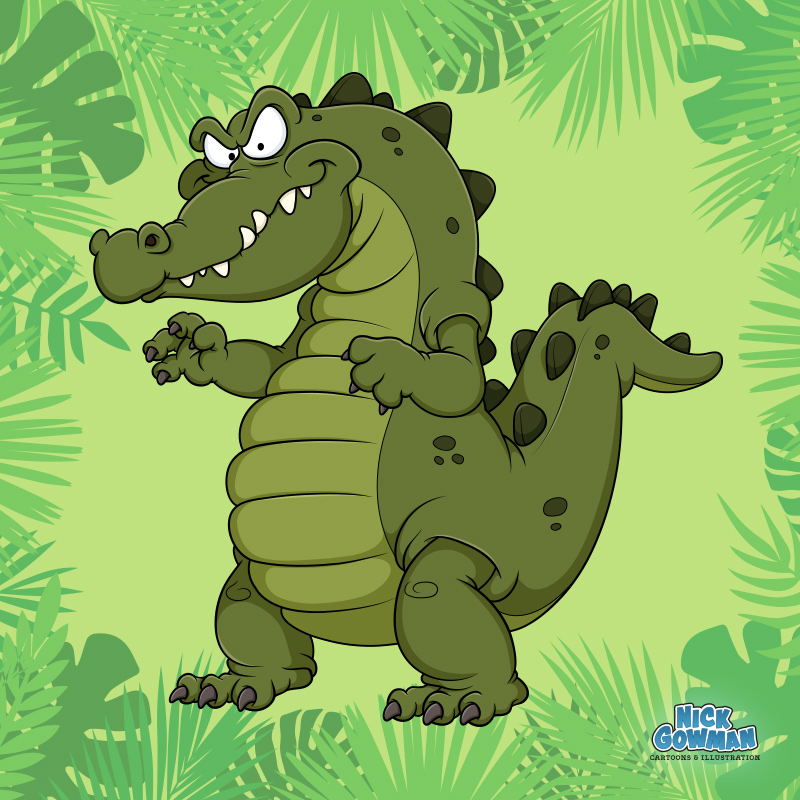This digital artwork showcases an anthropomorphized cartoon character striking a menacing pose. The character resembles a dinosaur or alligator, predominantly dark green with a lighter green belly. It stands upright on its hind legs, with a human-like posture, and has distinctive white eyes with black pupils and a long, crocodile-like mouth revealing sharp white teeth. The creature's body features darker gray spots and triangular, rock-like horns along its back. Its hands and feet are equipped with purple, sharp nails, and it sports a long tail. The background is a light green hue, accented by a border of darker green tropical leaves. In the bottom right corner, text in blue reads, "Nick Goldman."